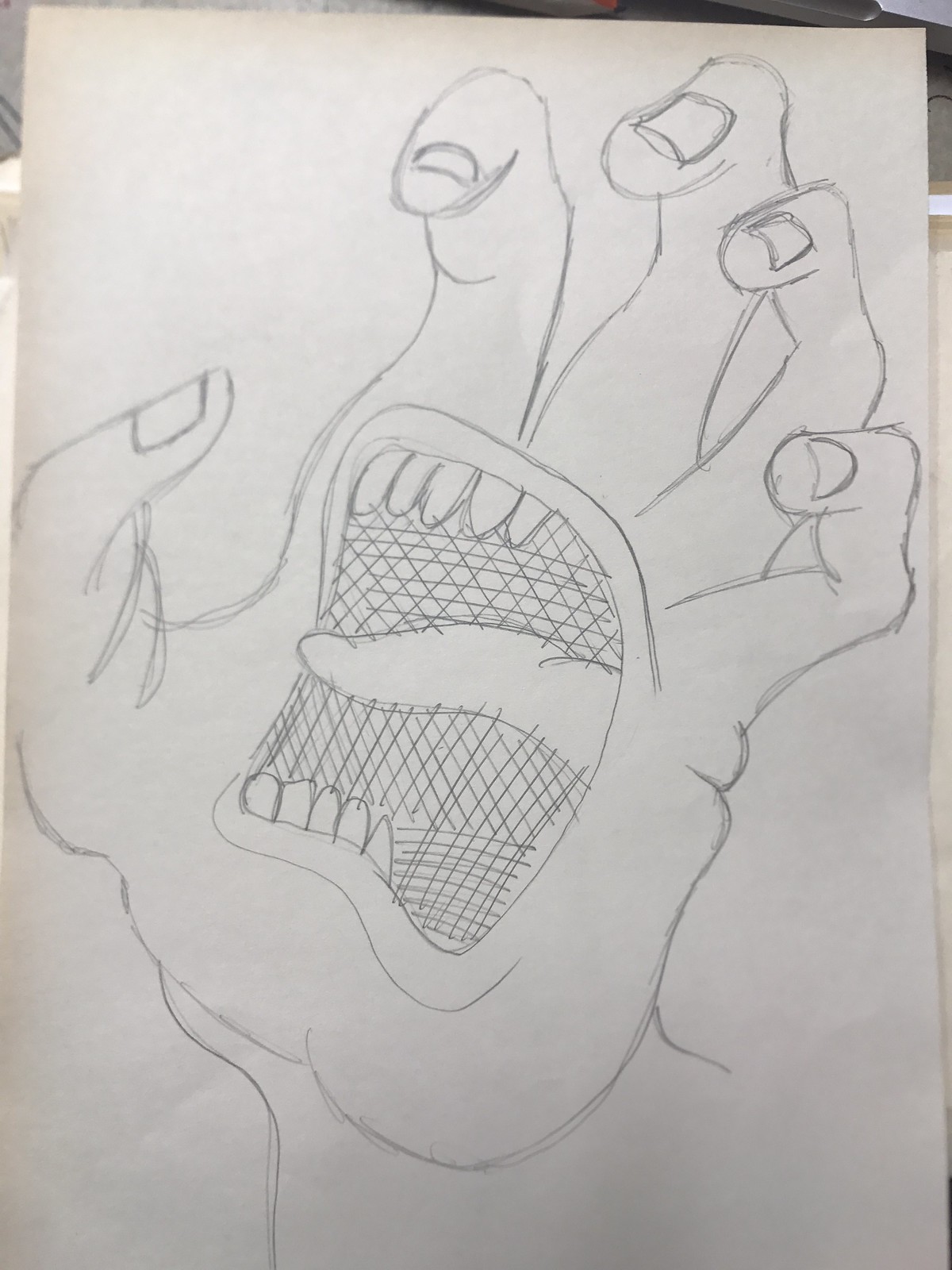This photograph showcases an intricate pencil drawing of a monstrous hand, expertly sketched on a white sheet of paper. The primary focus of the drawing is a human hand with grotesque, monster-like features. The palm of the hand is transformed into a large, gaping mouth filled with rows of razor-sharp teeth, with an elongated, menacing tongue hanging out, creating an impression of it screaming or issuing a battle cry. The fingers are adorned with what appear to be eyes on stalk-like structures, with the fingernails possibly doubling as these eerie eyes, enhancing the surreal and nightmarish quality of the hand-face hybrid. The drawing is held in the upper left corner by a visible hand, placed against a light wooden desk in the background, adding context to the framing of this striking image.